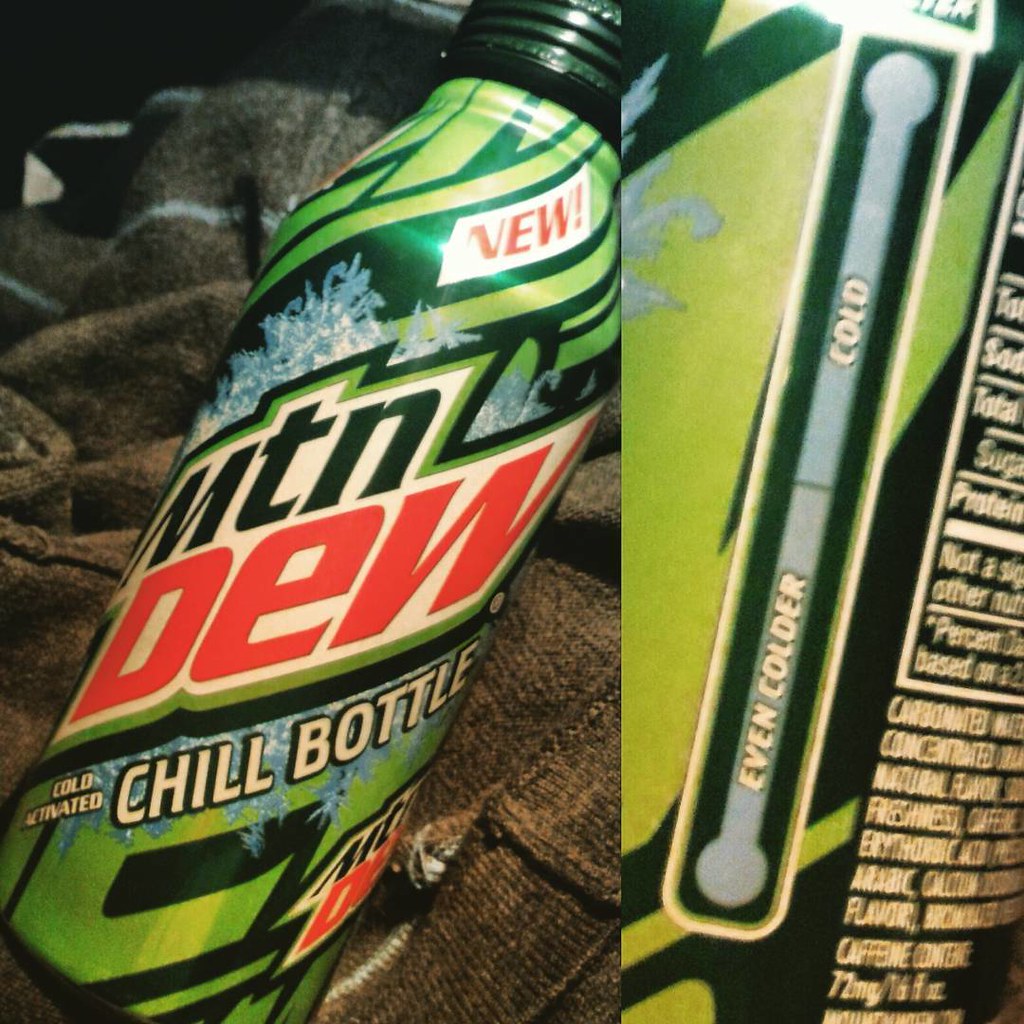This image consists of two side-by-side close-ups of a vintage Mountain Dew bottle, likely over 15 years old, showcasing its distinct "cold activated chill bottle" feature. The left side displays the full bottle reclined on what appears to be a gray sweatshirt or towel, with hints of blue stripes suggesting a blanket or shirt in the background. The bottle prominently features the Mountain Dew logo with the "MTN DEW" text, and just below it, the phrase "cold activated chill bottle." Above the logo, the word "new" is boldly emphasized in red letters with an exclamation mark. The right side of the image provides a zoomed-in view focusing on a thermometer graphic on the bottle, marked with "cold" at the top and "even colder" toward the bottom. This close-up also partially reveals the nutritional information, including caffeine content and ingredients like total sugars and protein.